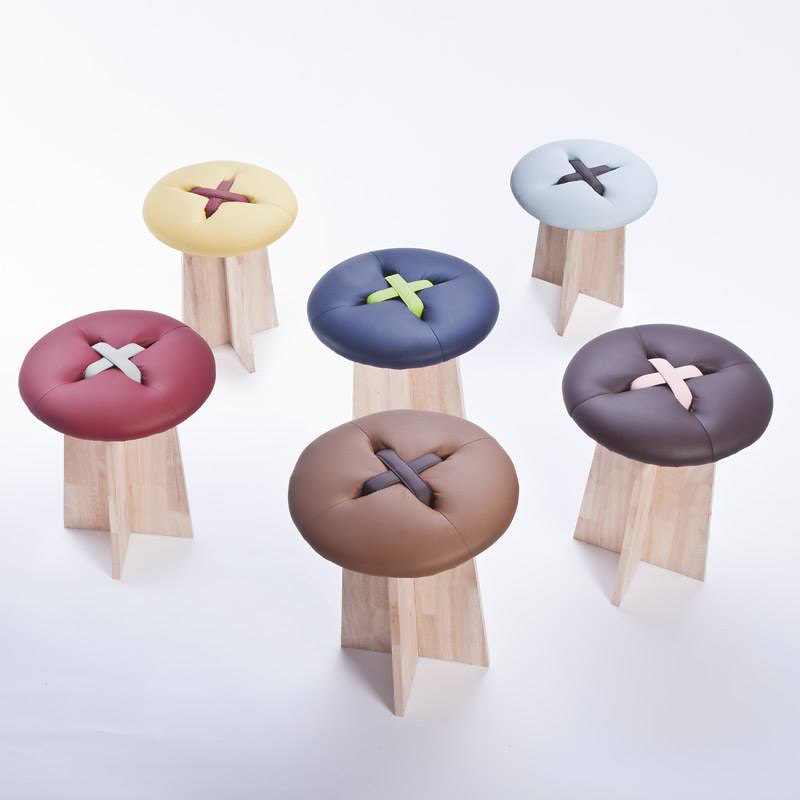The image displays a set of six distinct, stool-like figurines set against a completely white background, making it challenging to gauge their size. Each figurine features a base made of three crisscrossed wooden pieces, ensuring stability. The bases are crafted from light-colored wood. Atop each base, there is a circular, cushioned seat designed to resemble a button, featuring four holes with crisscrossed straps connecting them in an X pattern. The seats come in various colors with contrasting centers: one has a red seat with a white center, another is yellow with a brown center, a third is blue with a light green center, a fourth is light brown with a dark brown center, a fifth is pale blue with a dark gray center, and the last one is a darker brown with a tan center. The intricate detailing and diverse colors suggest an artistic or decorative purpose, although their exact function remains ambiguous.